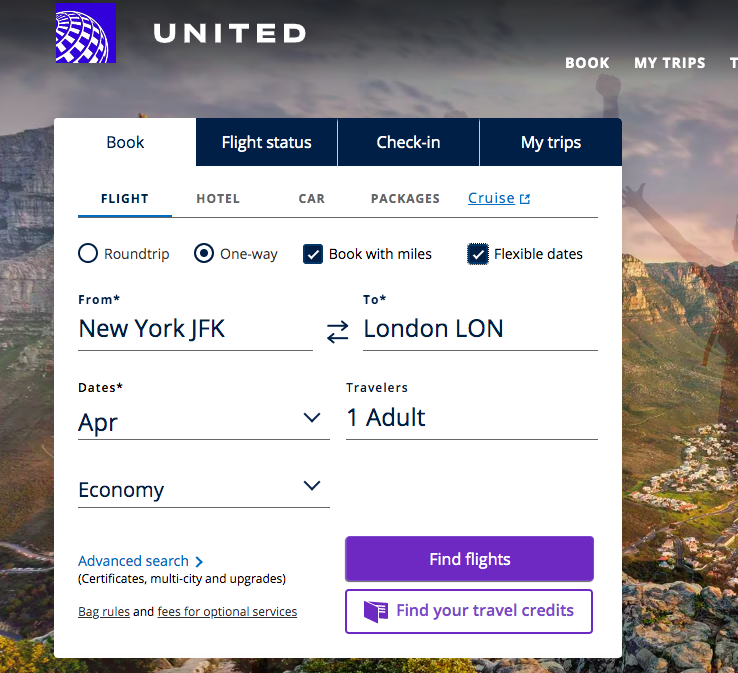The image is a square screenshot of the United Airlines homepage. In the upper left quadrant, "United" is prominently displayed in bold, white, capital letters. Adjacent to this text on the left is the United Airlines logo featuring a spinning globe on a blue background.

At the center of the screen, there is a white search box where users can input their information. The background of the homepage features a translucent image of a picturesque mountainous valley, adding a serene visual element. A silhouette of a person with their hand out is visible on the right side of the screen.

Two headers, "Book" and "My Trips," are visible at the top. At the center of the screen is a pop-up box with four selectable categories: "Book," "Flight Status," "Check-in," and "My Trips." The "Book" category is highlighted, with the term "Flight" underlined.

The search criteria indicate that the user is looking for a one-way flight booked with miles and flexible dates, traveling from New York (JFK) to London (LON). The selected month is April, and the travel class chosen is Economy. The search is set for one adult passenger. Beneath the Economy class option, a light blue link for an advanced search is available.

At the bottom right of the pop-up box are two buttons. The purple button on the left reads "Find Flights," while the white button with purple text on the right reads "Find Your Travel Credits."